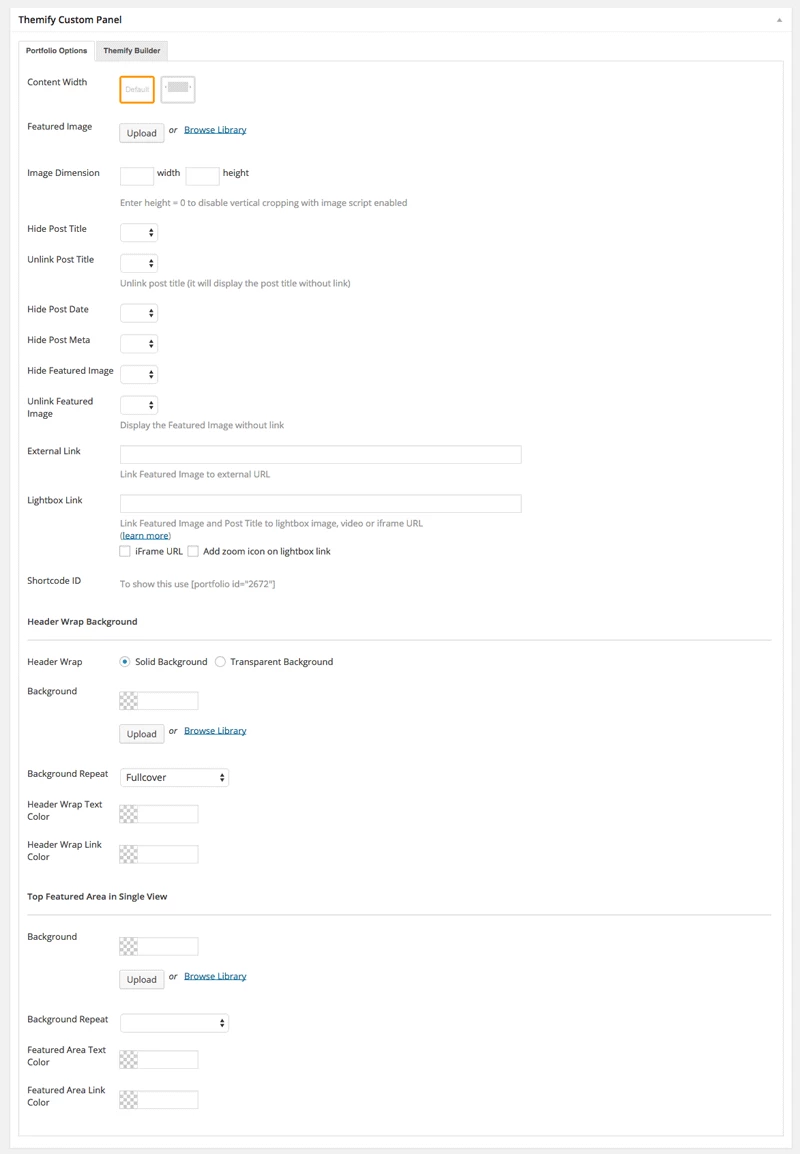The image showcases the Themephy Custom Panel interface. Set against an all-white background, the interface appears compact and requires closer inspection to read its details. At the top, there is a search bar followed by a smaller gray bar and a slightly lighter white bar labeled "constant width." An orange-outlined square and a plain square are also present.

Additional elements of the interface include labels such as "Featured Image," "Upload Image," and "Dimension." Checkboxes for options like "Hide Post Title," "Unlinked Post Table," "Hide Post Date," "Hide Post Meta," "Hide Featured Image," and "Link Featured Image" are visible but are all empty and unselected. Each checkbox is accompanied by arrows pointing upwards and downwards.

Below these sections, there are long input boxes intended for user-provided information. The entire interface is divided into three sections: a larger section at the top and two smaller sections beneath it. Sporadic letters in blue, indicating clickable links, are scattered throughout the interface.